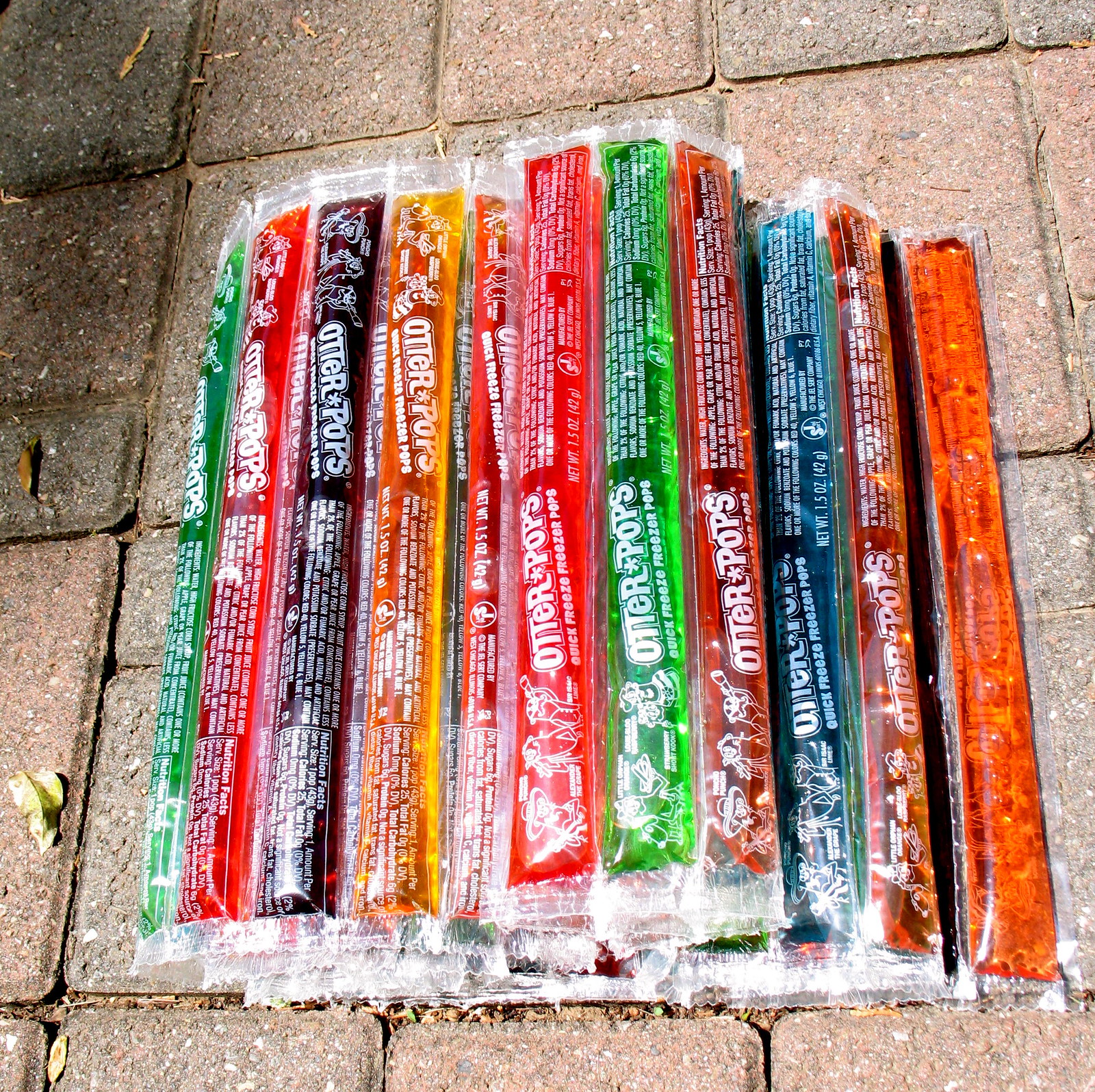A detailed and descriptive caption based on the input:

A photograph captures a pile of colorful, unfrozen Otter Pops laid out on a brick-paved ground. These popular summer treats, typically frozen to provide a refreshing snack, are currently liquid-filled in their clear plastic tubes. The Otter Pops are seen in a spectrum of colors including red, green, yellow, orange, blue, and purple. Each tube features the brand name "Otter Pops," along with two otters, the text "Quick Freeze Pops," and the net weight of 1.5 ounces (42 grams). The brick pavers beneath, a mix of dark gray and light brownish-red, show visible gaps with remnants of sand and fallen leaves in various stages of decay. The left side of the image features additional leaves in shades of light brown and green, emphasizing the outdoor setting.